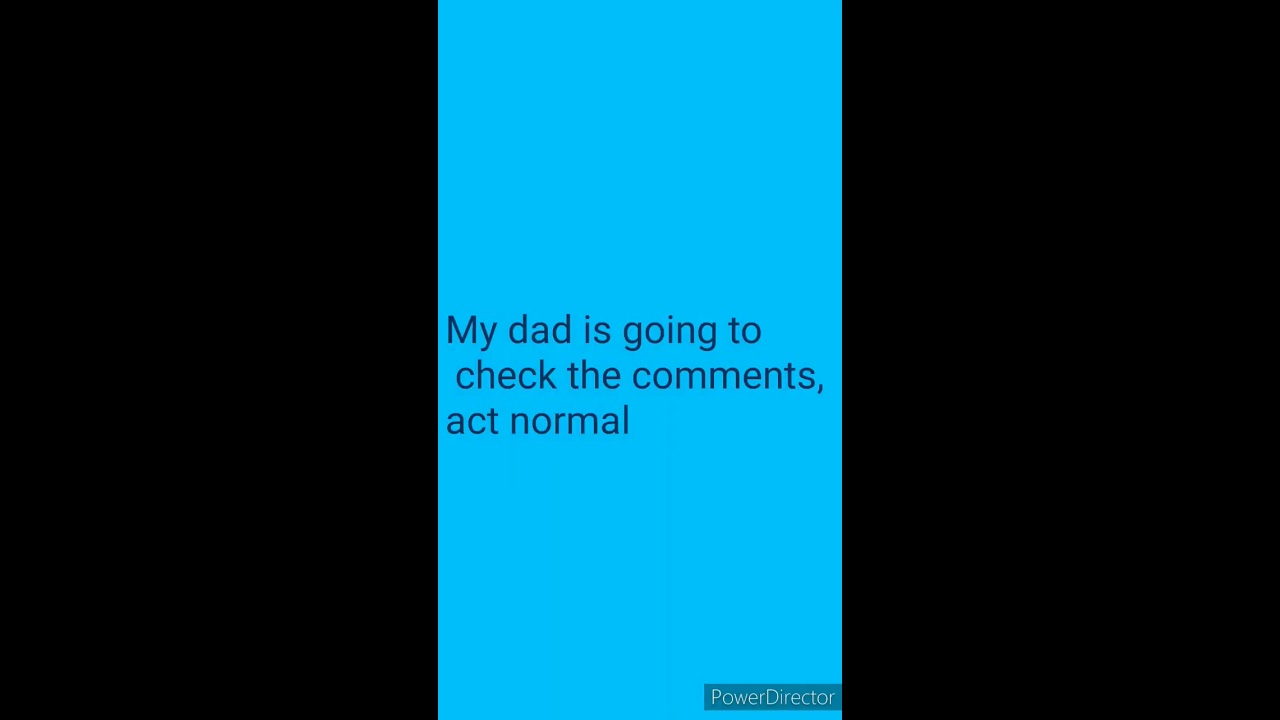The image features a vertically oriented rectangle with a light blue background. In the center, there is a dark navy caption that reads, “my dad is going to check the comments, act normal,” with a capital 'M' at the beginning and a comma after "comments." Towards the bottom right corner, there is a small, light gray box containing the manufacturer's label, "PowerDirector," in white text. The overall layout is divided into three sections: the blue central portion flanked by equal-sized black sections on the left and right. Additionally, the image includes a small thumbnail icon in the top left corner, depicting a failed image load with a green lower left and a blue upper left corner, complete with a white circle and a diagonal white bar extending from the bottom center to the middle right edge.